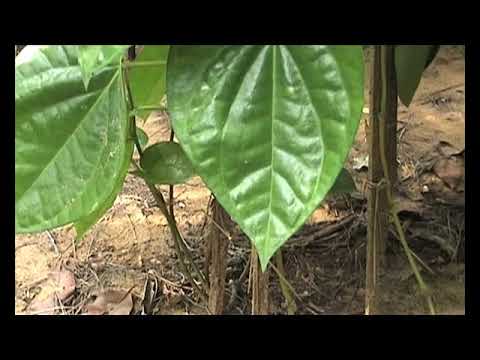The image depicts an outdoor scene with a barren, hardened soil area, devoid of other vegetation. Emerging from this crusty ground are three tall, woody-stemmed plants, supported either by string or posts to maintain their vertical alignment. In the lower right portion, the plants display large, bright green leaves with distinct veining, teardrop-shaped and shiny, suggesting a healthy, vibrant state. The leaves are prominently situated in the foreground and occupy significant portions of the left and middle areas of the frame. The soil beneath appears packed down and is interspersed with some stray twigs, but otherwise remains bare. The photograph is noticeably sunlit, enhancing the vivid green of the plant leaves against the monochromatic brown soil. The image is cropped within a black border, focusing on the stems and the lush lower leaves while the tops of the plants are not visible.